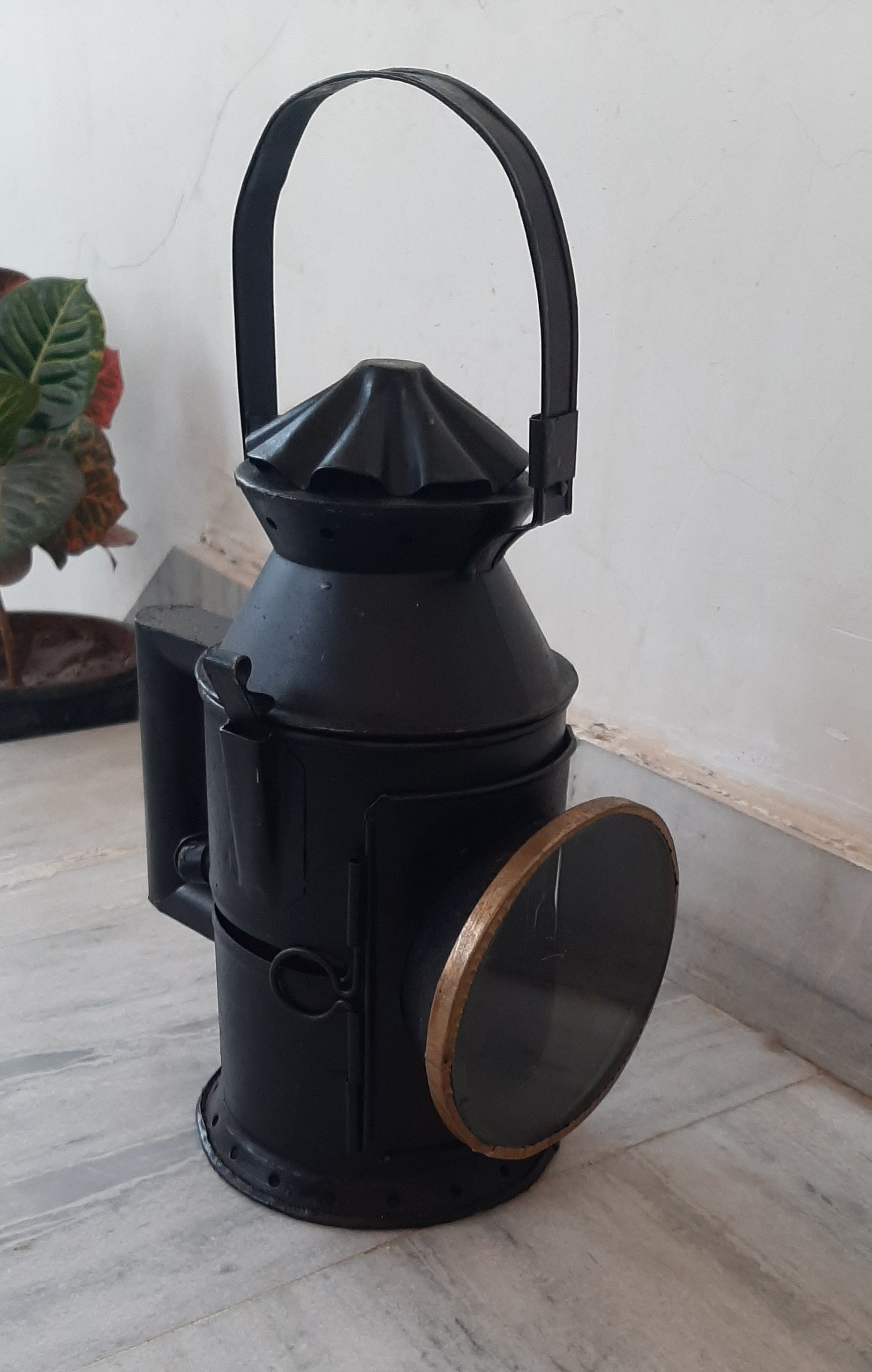The image depicts a black, lantern-like canister with a cone-shaped top, reminiscent of an old-school fire hydrant, sitting on an interior floor. The canister features a large black handle and a circular glass window with a gold or copper trim on the front, possibly for viewing or illuminating the contents. This glass window is framed with a ring, hinting it might function as a door. The object is positioned on either a linoleum, ceramic tile, or marble-like floor, which looks dingy and dirty, particularly on top. In the background, there's a gray wall with darker trim and a picture or actual view of a green plant with large leaves, some of which have red and brown hues. The canister is clearly movable, as suggested by its various handles and latches, but its exact purpose remains ambiguous.